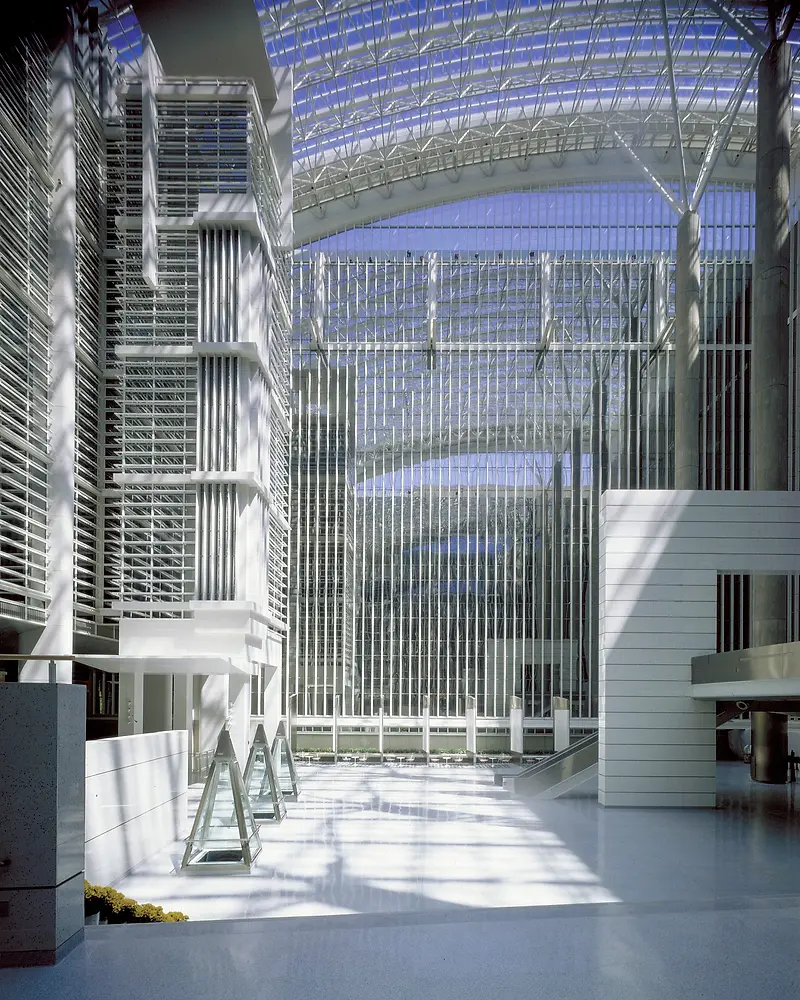The photo captures the expansive hall of a towering building, characterized by its remarkable height that nearly conceals the ceiling from view. The ceiling of this grand structure is transparent, composed of large glass windows that allow ample sunshine to flood the open space below. The walls and floor are uniformly white, enhancing the pristine and airy atmosphere, while certain elements, like metal accents and a steel ramp on the right, break the monochrome with a sleek silver finish. The right side also features a staircase adding to the sense of verticality. Dominating the scene are statues shaped like triangular prisms, adding an artistic touch. The overall ambiance suggests that the space could be a museum owing to its immense size and modern aesthetics. However, the design could also be reminiscent of a shopping mall or even an atrium, providing a versatile setting where natural light is a key feature. The blue sky is visibly clear through the glass ceiling, complementing the indoor structure's openness and airy feel.